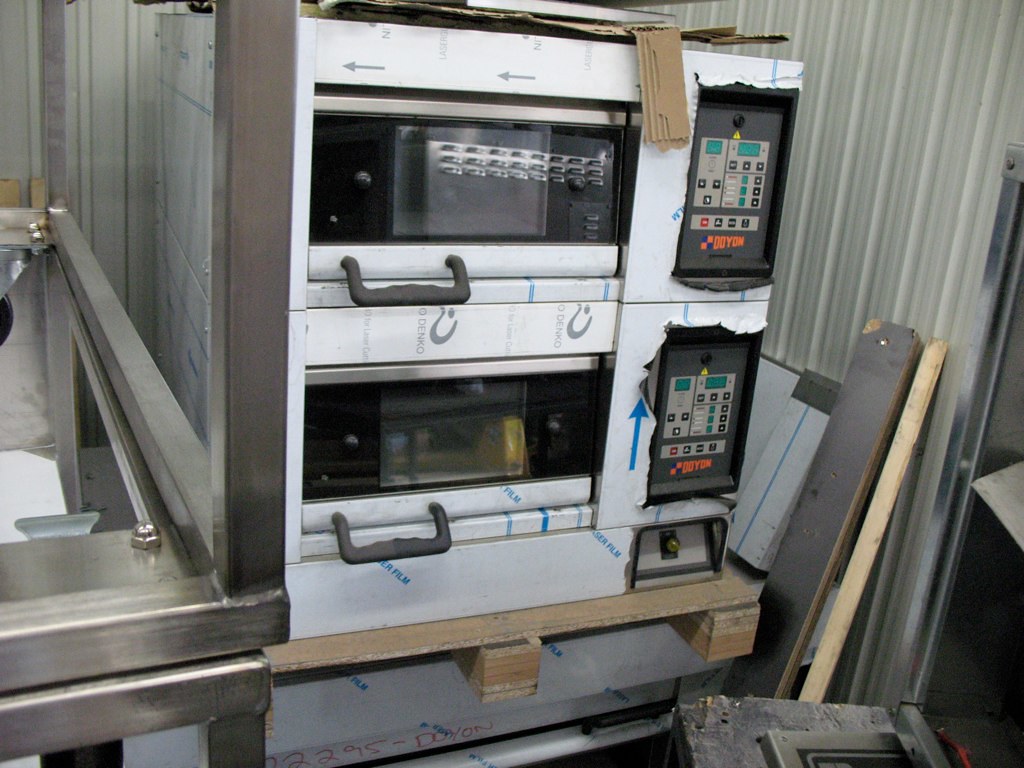The photograph depicts a pair of large industrial ovens, stacked one on top of the other, situated in what appears to be a warehouse setting with a light gray backdrop. The units are predominantly silver and enclosed in a protective white, gray, and blue film, indicating they are newly installed but not yet unwrapped. Each oven features a dark gray handle and a clear glass viewing window, complemented by a push-button control panel located on the right side of the units. The control panels also contain small screens and a key insertion point to presumably activate the machines. The brand name "Doyon" can be seen in orange beneath the control panels.

The ovens, likely designed for heavy-duty cooking tasks such as roasting large items or baking pizzas, are resting on a wooden pallet amidst various wood scraps and cardboard, suggesting an ongoing installation process. To the left side of the frame, there is a brushed stainless steel shelving unit. The surrounding area is cluttered with more construction materials and packaging, reinforcing the impression that the setting is currently under assembly.